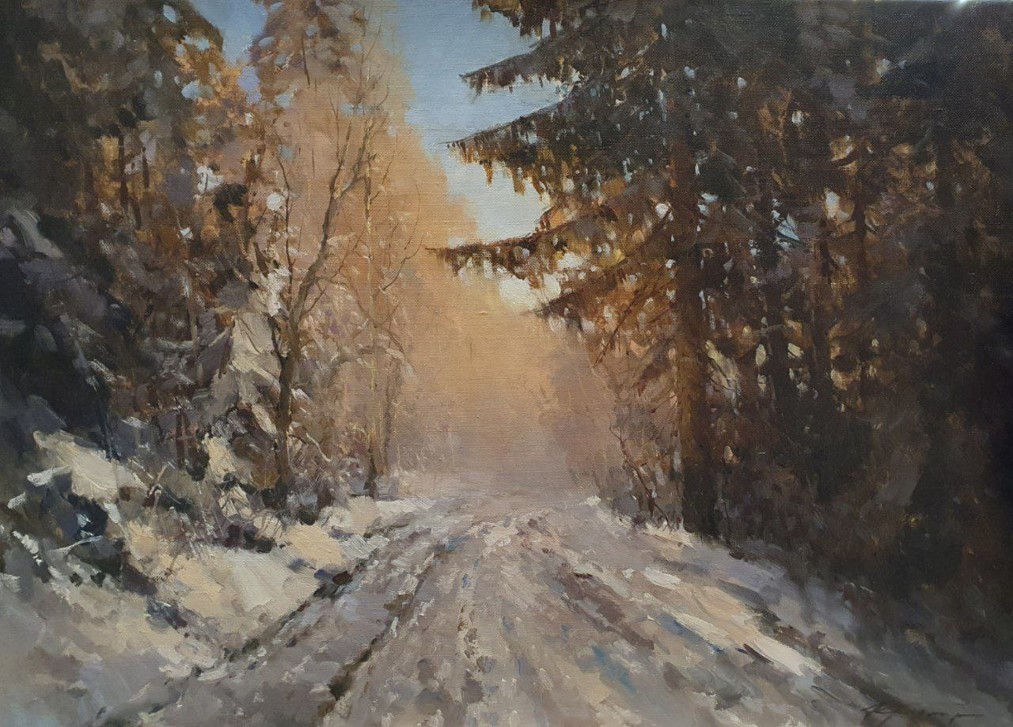This full-color oil painting, rectangular with a longer horizontal edge, features a serene winter landscape of a mountain road meandering through a forest. The scene is painted in a somewhat blurry style, with muted colors predominating the composition. The road, appearing grayish-white and covered in slushy tracks, leads from the left towards the center, gradually fading into a misty background. On either side of the road, a variety of trees are depicted—evergreens with snow-laden branches, coniferous trees primarily on the right-hand side catching the sunlight, and some deciduous trees with darker, slightly yellow leaves. The trees exhibit a mix of green and brown hues, with patches of snow adding a stark white contrast, particularly heavier on the left side. A touch of blue sky peeks through the treetops, enhancing the tranquil, wintry ambiance of the forest.